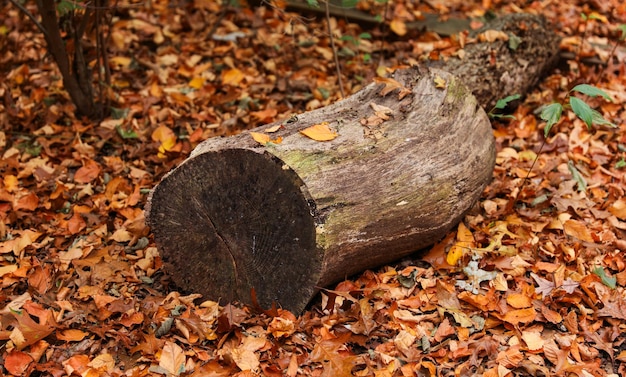This photograph captures a professionally-taken, well-lit image of a cut tree stump lying on its side amidst a forest floor covered in autumnal foliage. The inside of the tree is exposed, showcasing where it was sawed, likely with a chainsaw, suggested by its straight, flat face. The outer bark of the log appears weathered and has patches of white and moss, indicating age and decay. The environment around the stump is a mosaic of colorful, decaying leaves in hues of rusty orange, tan, brown, and some splashes of yellow and red, suggesting the setting is during the fall season, potentially on the East Coast between October and November. The scene evokes a sense of a natural, undisturbed woodland, possibly along a hiking trail, with the log and a smaller decaying log nearby, not arranged for practical use but rather left to nature’s course. There is no text in the image, enhancing its serene, untouched quality.